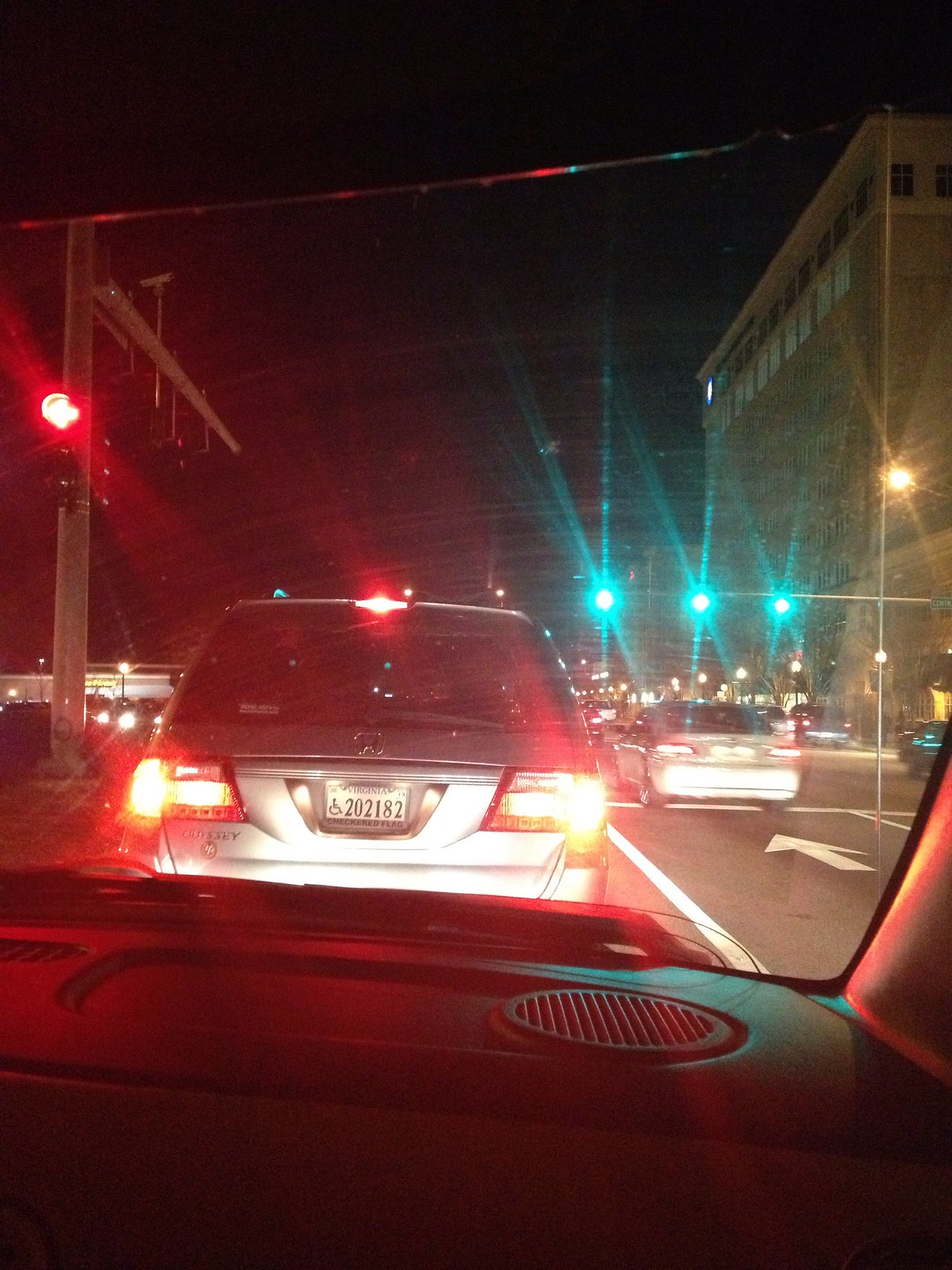The image captures a nighttime scene from inside a vehicle, looking out onto a two-lane road. Multiple cars are ahead on both lanes, amidst a backdrop of numerous lights illuminating the scene. Eye-catching beams of blue light emanate from the right side while a single, vivid red light glows on the left. On the right side of the road stands a tall building. The road itself is made of asphalt, marked by a white arrow on the right side, indicating the direction of traffic. The sky is a pitch-black canvas, interspersed with the glare of headlights and streetlights, creating a surreal blend of red and blue beams piercing through the darkness.